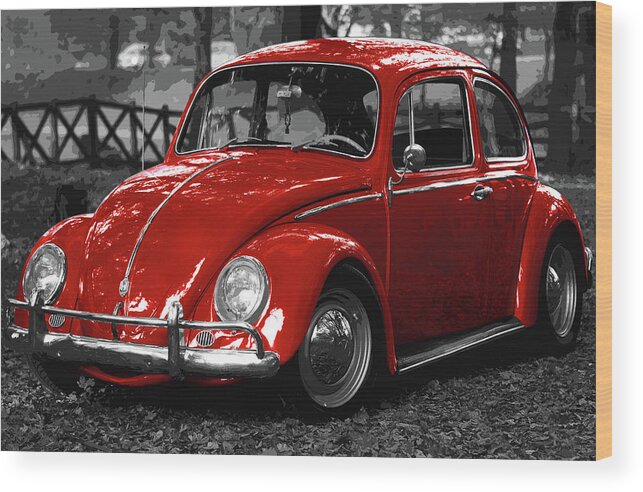The image captures a striking, bright red Volkswagen Beetle, possibly an early 1960s or original model, centered prominently against a black-and-white background. The Beetle gleams with its shiny cherry red paint while the rest of the details, including the chrome bumper, wheel covers, dual headlights, side mirrors, and door handles, remain in a monochrome palette. The car is set on a textured, leafy ground, suggesting an outdoor setting, and is facing towards the left-hand corner, as if ready to drive off. Behind the Beetle, the background features a somewhat stylized and pixelated nature scene, revealing chunks of trees and a wooden fence with crosshatched patterns, though these elements blur in comparison to the sharply focused vintage car. The interior of the Volkswagen, like its exterior details aside from the paint, retains the black-and-white theme, further emphasizing the car's vivid color.